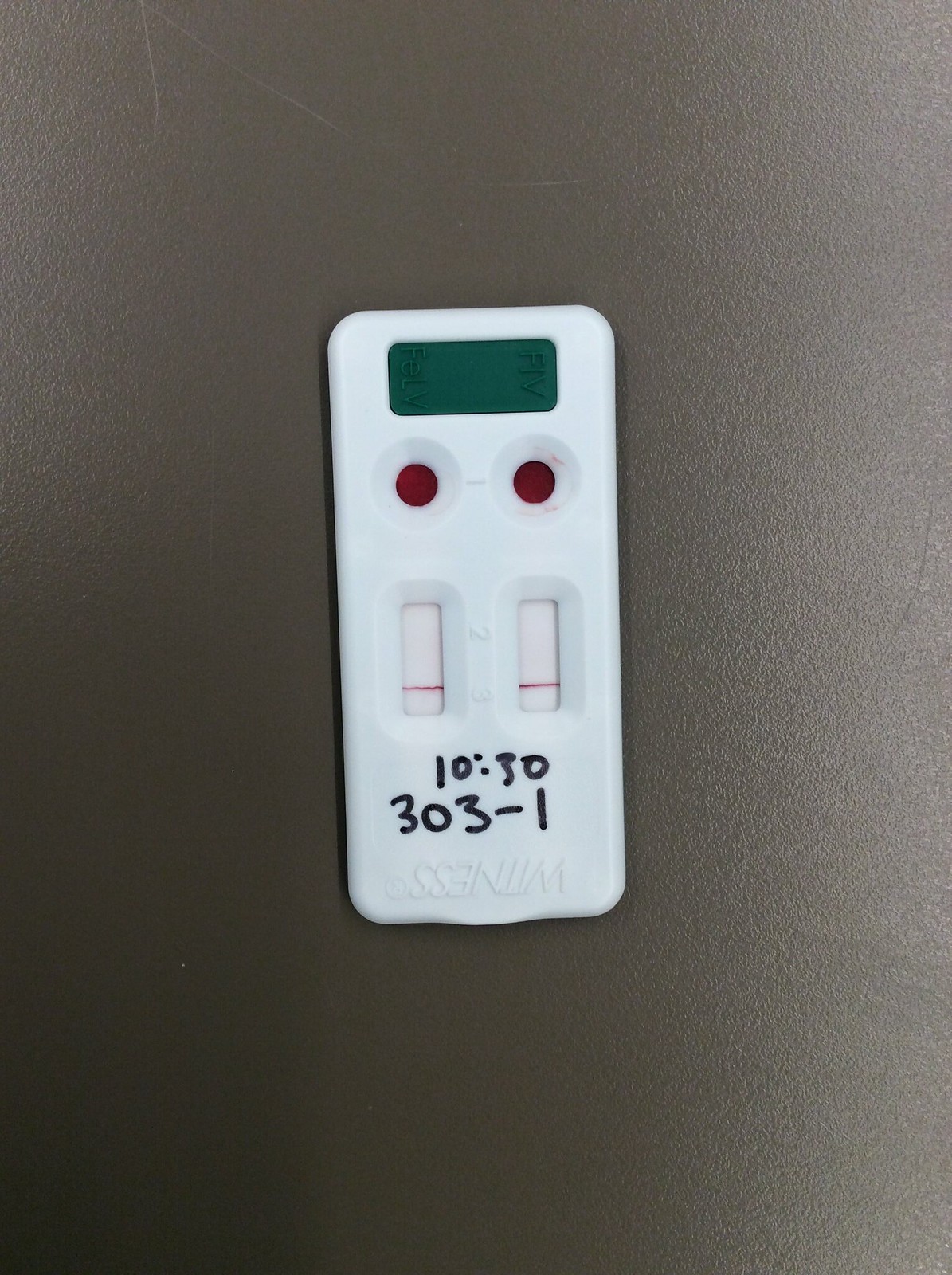The image presents a COVID-19 home test kit placed on a gray surface, which could be a table. The test kit is branded with the name "WITNESS." The kit features multiple windows, each designed to display the test results. Notably, each window shows one clear red line, indicating that the test has been administered and the results are available. Additionally, a small red dot is visible. The labeling includes "303-1," "1030," and "FIV-FELV," suggesting it could be a hybrid diagnostic tool. The presence of clear results in the windows, combined with the distinct red lines, indicates that the test has provided definitive results.